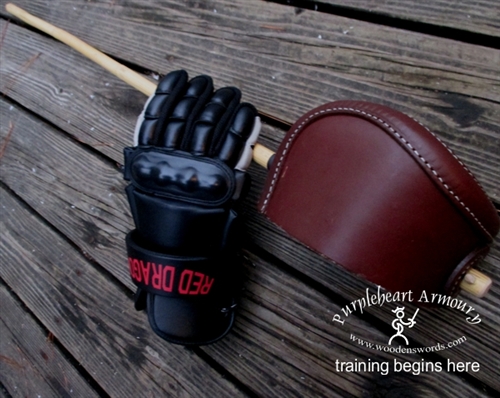The image shows a black leather fencing glove with red text that reads "Red Dragon." The glove is positioned as if gripping a beige-colored fencing post, which features a red burgundy leather guard with white stitching. These items rest on a brown, weathered wooden surface, resembling a picnic table. In the bottom right-hand corner, there is a logo for Purple Heart Armory, accompanied by the text "Training begins here" in lowercase letters. An image of a stick figure fencer wielding a sword, along with the website "www.woodenswords.com," is also visible. The glove's design includes armored knuckles for protection, indicating its use in fencing practice.